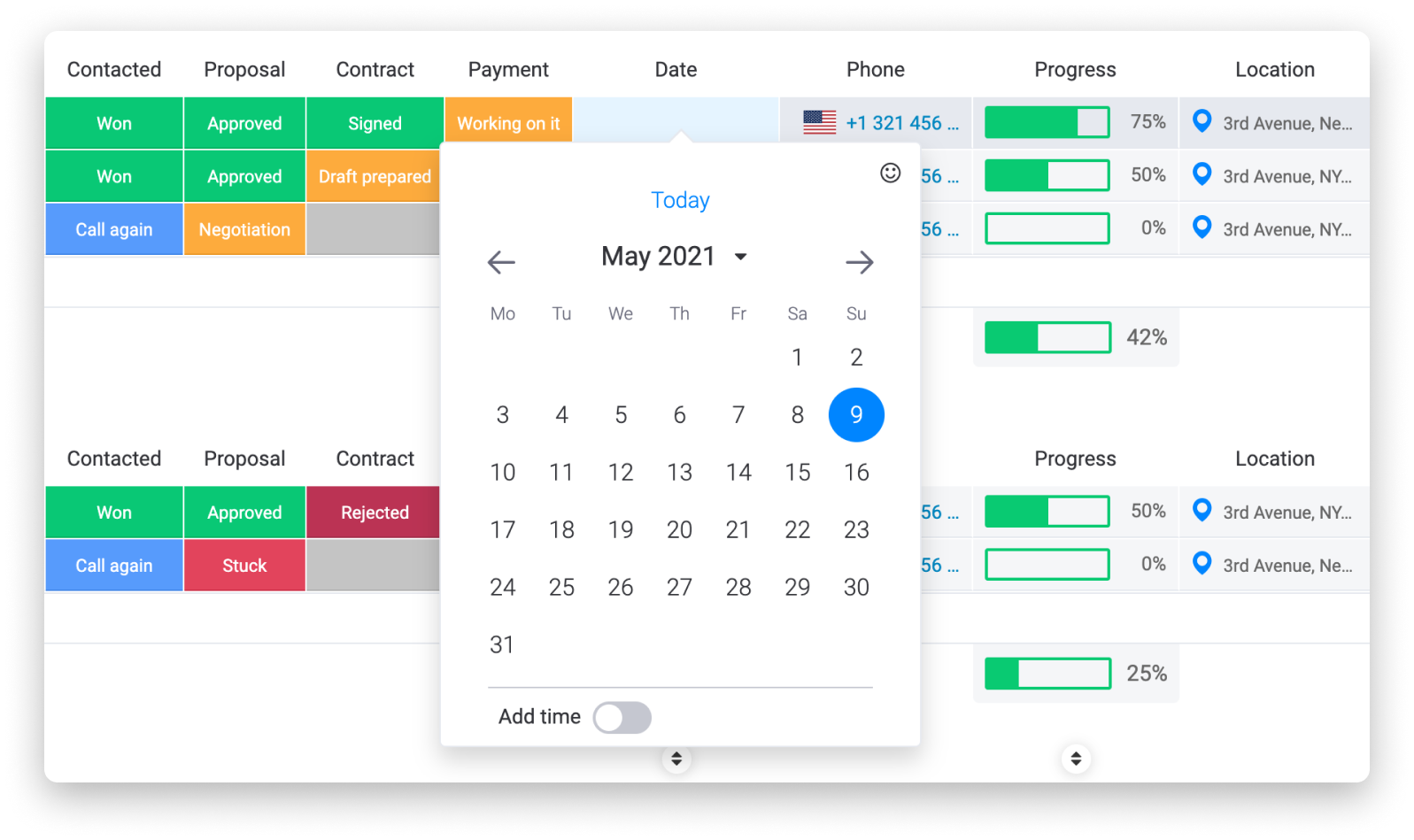The image depicts a screenshot of a business tracking software interface, featuring various sections and tools aimed at managing client interactions and project progress. The background displays a series of labeled categories, including "Contacted," "Proposal," "Contract," "Payment," "Date," "Phone," "Progress," and "Location," suggesting the software is designed to streamline business operations and monitor client journeys.

Beneath this primary interface, additional status indicators are visible under categories like "Contacted," "Call Again," "Approve," "Proposal is Approved," "Negotiation," "Contract Signed," "Draft Prepared," and "Payment," likely representing different stages of client or project management.

Prominently overlaid on the main interface is a pop-up calendar for date selection, specifically showing May 2021. The calendar highlights the 9th of May, indicating that this might be the current date within the context of the screenshot. The detailed layout and comprehensive tracking options imply that the software is a robust tool for business professionals to manage and track their client deals and project timelines efficiently.